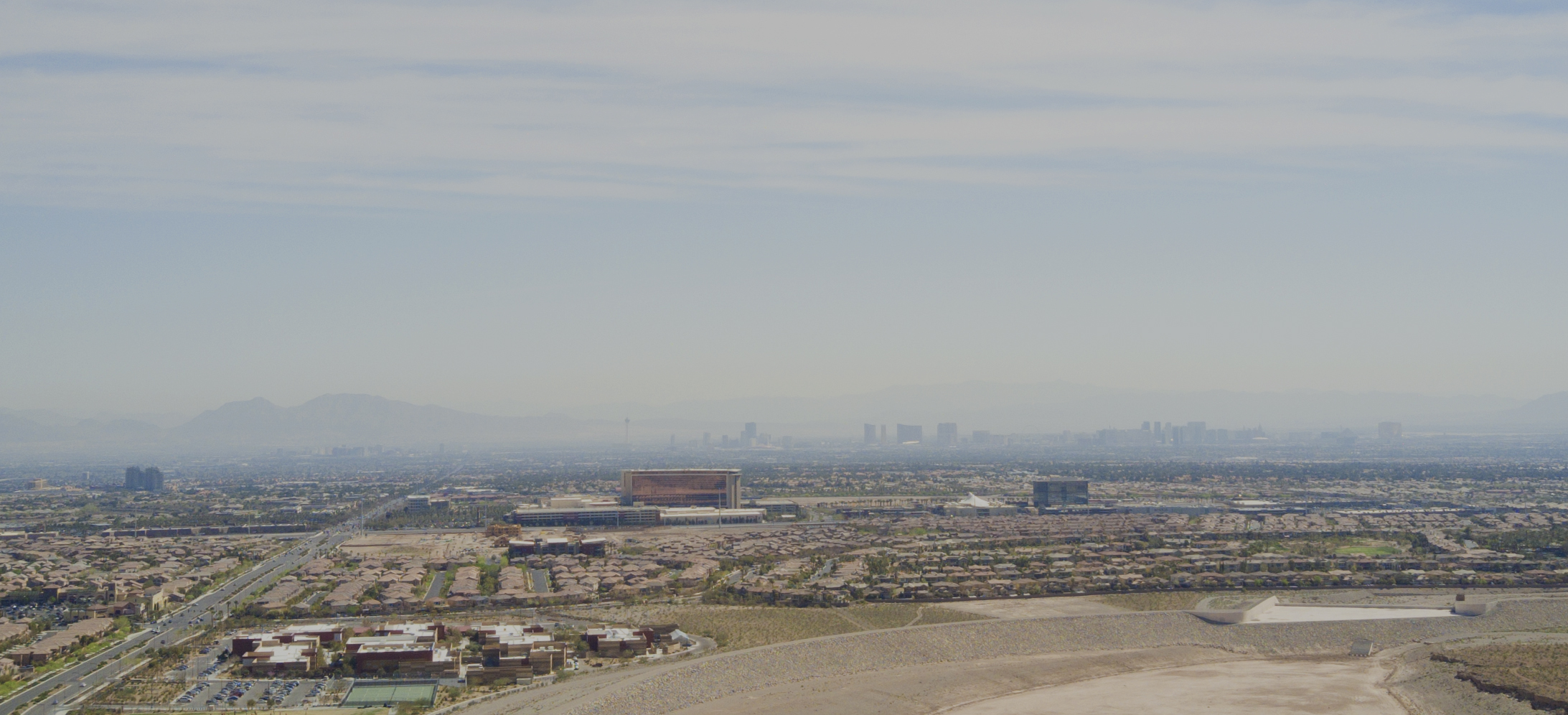The image, oriented in a landscape mode, captures an expansive aerial view of a serene cityscape or industrial area. The upper two-thirds of the photo depict a vast blue sky adorned with scattered clouds. This sky meets the horizon, delineating a clear line where the sky meets the distant terrain. Far off in the distance, faint outlines of mountains and buildings peek through, partially obscured by the haze, adding a sense of depth to the landscape.

In the bottom third of the image, a tranquil city or industrial area comes into focus. The lower left-hand corner reveals a network of roads or a freeway, indicating human activity and connectivity. Scattered throughout the scene are small houses and warehouses, suggesting both residential and industrial usage. Patches of green fields interspersed among the buildings hint at a blend of natural and developed land. The overall mood of the image is one of calm and quiet, with a harmonious blend of natural and urban elements.